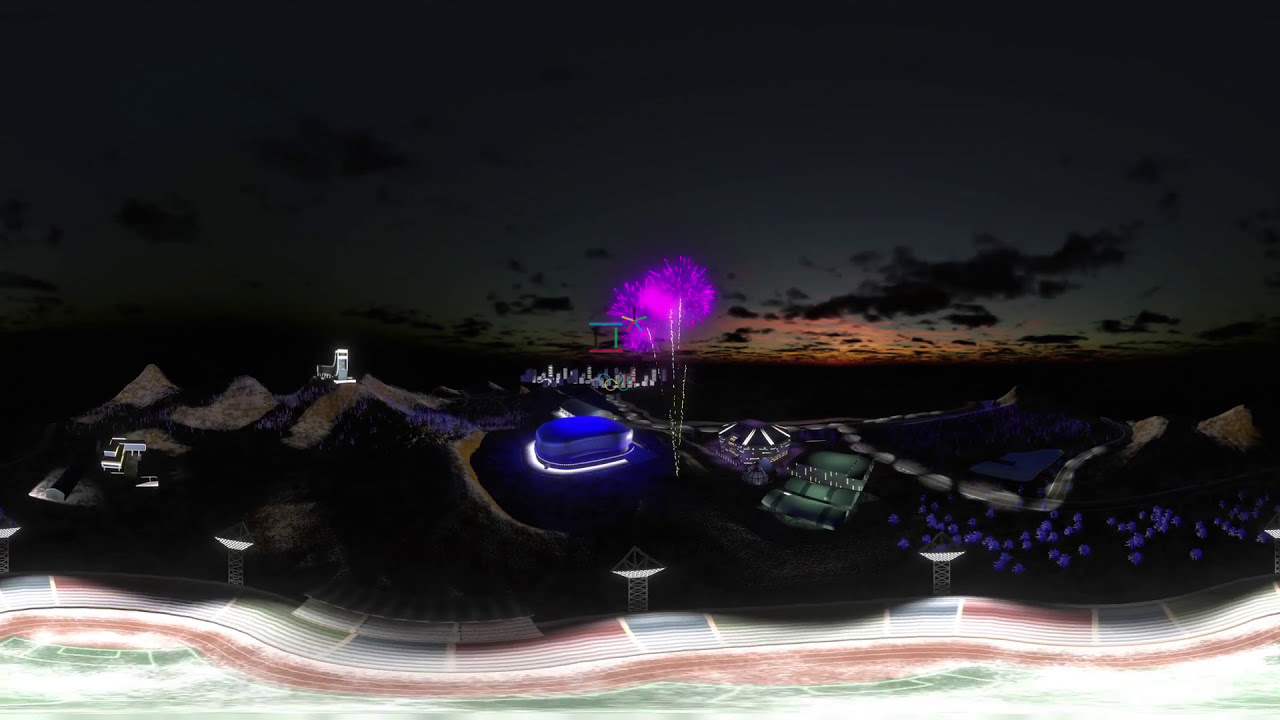In this highly distorted fisheye lens photo taken at night, the scene is bustling with vibrant activity reminiscent of an amusement park or a sports venue. At the very bottom, a light path streaks left to right with intermingling hues of green, orange, and white. Above this, dark pink and purple fireworks burst dramatically in the center, streaked with some light yellow trails. To the left, a round building is illuminated with a bright blue light atop it. On the right side of the fireworks, there's another circular structure with a black roof adorned with white lights, which appears to house a rotating carousel underneath. Nearby, a small green square resembling a miniature tennis court can be seen. Far in the distance, the horizon is tinged with the soft orange glow of a sunrise peeking through dark clouds, creating a striking contrast against the darkening sky. On the far right side of the image, small purple balloons add a whimsical touch. The entire scene combines the lively feel of a nighttime park with festive, colorful elements and distant cityscapes.